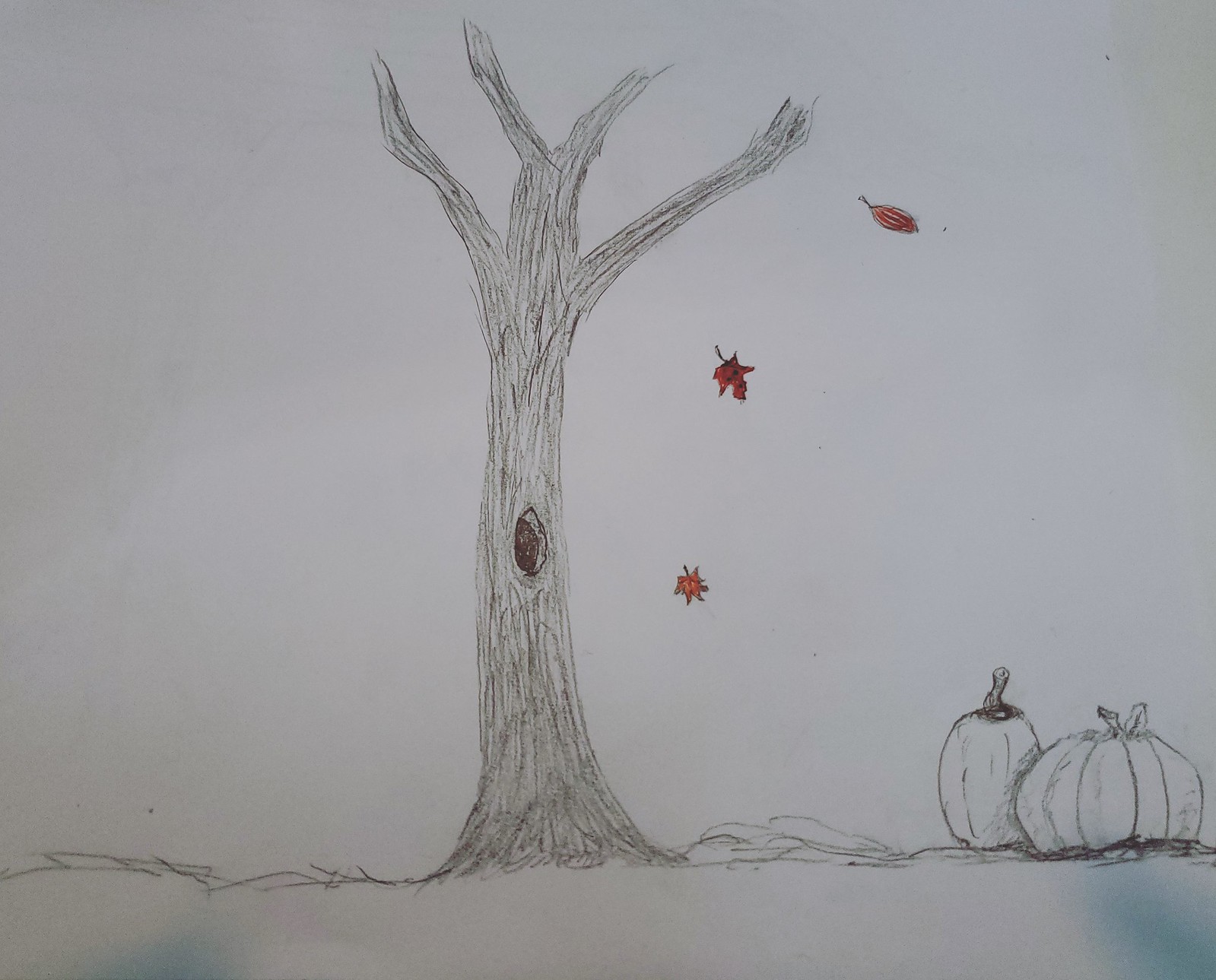A detailed bird's-eye view of a sketch rendered in pencil on white paper showcases an autumnal scene. Central to the image is a tree with a textured trunk featuring a shaded bark and a noticeable hollow in the middle. Positioned to the left of the pumpkins, the tree stands prominently in the center of the composition. Above the pumpkins, three distinct leaves fall gently to the right side of the tree. The leaves vary in design: a circular oval-type leaf, a red maple leaf resembling the Canadian flag, and another maple leaf with more spikes or offshoots colored in grey. To the far right, just before the border of the paper, two pumpkins rest side by side. One pumpkin is wide and circular, slightly overlapping the taller, thinner oval pumpkin to its left. Both pumpkins have detailed stalks, adding to the seasonal charm of the sketch.